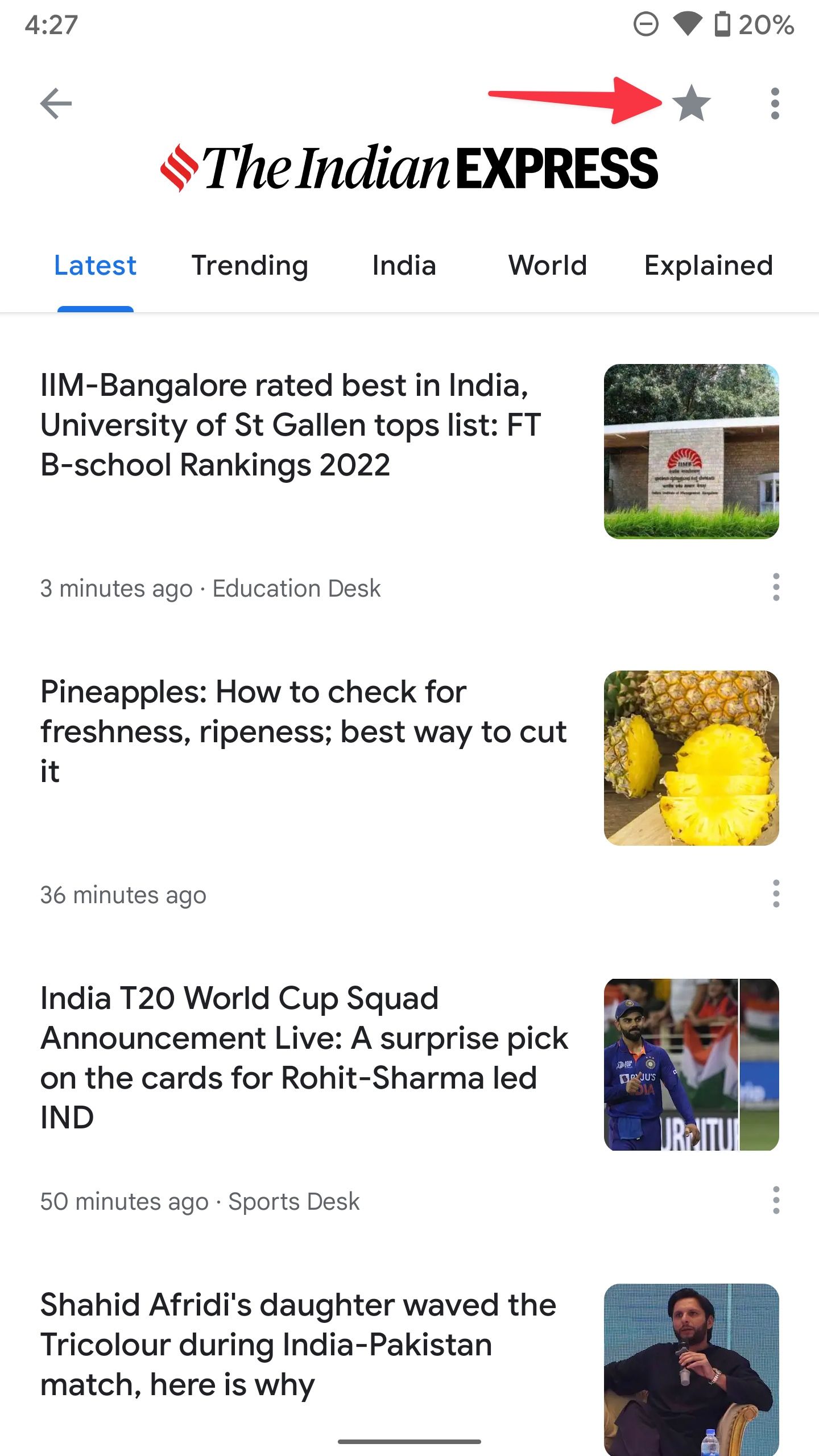The image features a white background overlaid on a smartphone screen. At the top, a filled red arrow points towards a grey star in the top right corner, which signifies a button to mark something as a favorite. Below the star, there is the text "The Indian Express" accompanied by an icon consisting of three red lines.

Underneath the newspaper title, there are several navigational tabs labeled "Latest," "Trending," "India," "World," and "Explained." The "Latest" tab is selected, highlighted in blue, while the rest are in black.

Further down the screen are various news articles arranged in a vertical list:

1. **First Article**: 
   - **Headline**: "IIM Bangalore, rated Best in India, University of ST, current top list, FTP school rankings in 2022."
   - **Details**: This article was posted three minutes ago by the Education Desk.
   - **Image**: On the right, there is an image of a university campus.

2. **Second Article**: 
   - **Headline**: "Pineapples: how to check for freshness, ripeness, best way to cut it."
   - **Details**: This article was posted 36 minutes ago.
   - **Image**: On the right, there are images of a whole yellow pineapple and a cut pineapple.

3. **Third Article**: 
   - **Headline**: "India T20 World Cup squad announcement live: a surprise pick on the cards for Rohit Sharma-led IND."
   - **Details**: This article was posted 50 minutes ago by Sports Desk.
   - **Image**: On the right, there is a picture of a cricket player.

4. **Fourth Article**:
   - **Headline**: "Saeed Afridi's daughter waved the tricolour during India-Pakistan match, here is why."
   - **Details**: There is no specific post time mentioned.
   - **Image**: On the right, there is an image of a person dressed in black sitting on a couch.

Each article is briefly described with its posting time and accompanied by relevant images on the right side of the text.